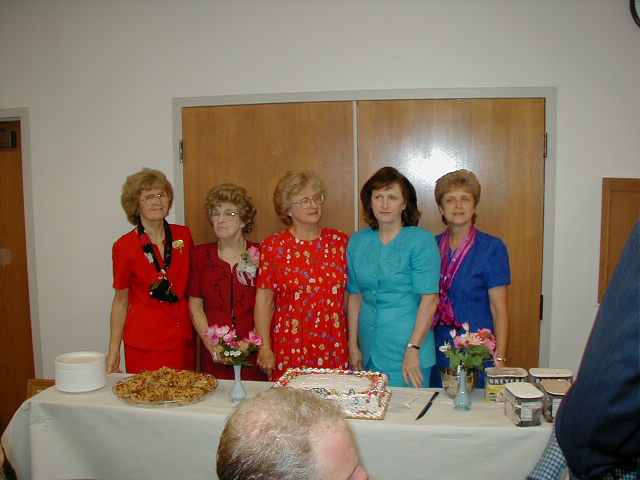This photograph captures five older white women standing closely together behind a banquet table, in front of a large double wooden door with white framing and additional white walls visible. The women, dressed in a mix of red and blue short-sleeved dresses with various designs and flower attachments, exhibit a range of pale skin tones and short hairstyles – four having blonde curly hair and one sporting longer dark brown hair. Three of the women are wearing large glasses with clear lenses.

The banquet table in front of them is elegantly covered with a white tablecloth and laden with an assortment of items arranged in a symmetric display. Central to the table is a large white cake adorned with decorated frosting. Flanking the cake are two vases filled with pink flowers and green leaves. To the left of the cake, there is a glass bowl or platter holding a brown food item, which might be cookies, as well as a stack of white paper plates. On the right side of the cake beside one of the flower vases, a knife is laid out. Further to the right, there are four large containers of Breyers ice cream, clearly labeled in white text, consisting of two vanilla and two chocolate tubs. The overall setup suggests a celebratory event, harmonized by the coordinated attire and symmetrical arrangement of food and decor.